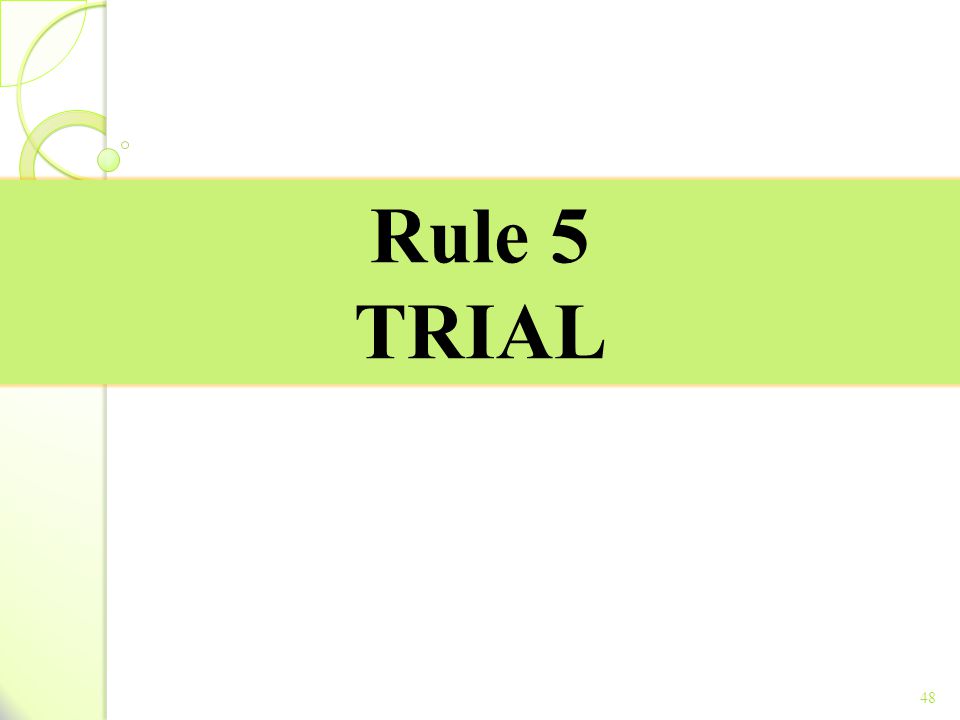The image features a prominently wide, lime green horizontal rectangular box at its center, set against a white background. Within this box, bold black text reads "RULE 5" with "TRIAL" written in all capital letters beneath it. To the left, there is a vertical light gray strip interspersed with blue. Positioned at the top of this strip is a series of shapes: a quarter circle outlined in lime green, next to a semi-circle also outlined in green, and beneath these, a smaller quarter-circle outlined in thick lime green. Additionally, at the lower right corner of the image, the number "48" is discreetly printed. The lime green rectangle features brown borders along its top and bottom edges.